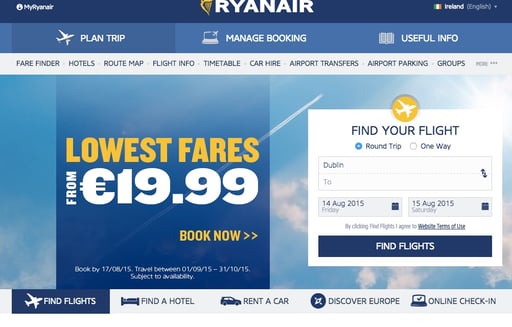The image showcases a section of the Ryanair interface. At the top, there's a dark blue header featuring a white user icon with a blue silhouette on the left, and the text "myRyanair" spelled out as "R-Y-A-N-A-I-R" on the right. In the middle of the header, there's a gold harp logo, adjacent to the word "Ryanair" written in bold, white, boxy capital letters with no spaces. 

On the right side, the Irish flag is displayed, accompanied by the word "Ireland" in lowercase bold white letters, followed by an indication that the interface is in English.

Below this, there's another blue header with menu options. The leftmost option, which is selected, has a darker blue background and features a white plane icon with the text "PLAN TRIP" in white uppercase letters. To the right, there are two more options with lighter blue backgrounds indicating they are not selected. The middle one displays a laptop with an airplane coming out of the top right corner, labeled "MANAGE BOOKING" in bold white capital letters. The next option shows an open book icon, labeled "USEFUL INFO" in similar white capital letters.

Beneath this, a white strip houses a series of menu options listed in black capital letters. The options are: "FAREFINDER," "HOTELS," "ROUTE MAPS," "FLIGHT INFO," "TIMETABLE," "CAR HIRE," "AIRPORT TRANSFERS," "AIRPORT PARKING," and "GROUPS." At the end, there is smaller gray capital text "MORE" followed by three gray dots, suggesting additional options are available upon clicking.